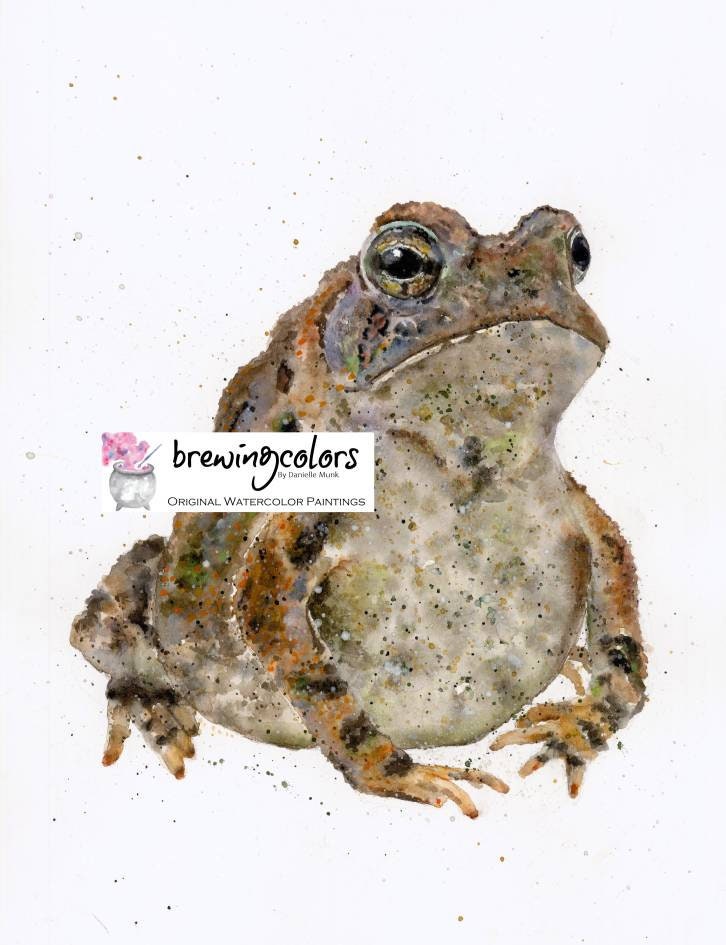The image is of a vibrant and detailed watercolor painting by Danielle Monk, vividly portraying a toad. The toad is positioned centrally, its body angled slightly to the right while its face looks directly forward. It has a white belly with mottled brown and black skin, and its large eyes are brown with black centers. Its front legs, with visible claws and webbed feet, are prominently displayed, with the left front leg slightly more visible. The back legs, particularly the left one, show the four toes clearly, while the right back toes are only partially visible.

The setting of the painting features a white background with subtle specks of paint splattered in various areas—brown specks in the upper left corner and greenish-brown specks below.

Overlaying the painting, about two-thirds down on the left side, is a horizontally oriented white rectangle. Inside this rectangle is the logo for "Brewing Colors, Original Watercolor Paintings" in black lettering. To the left of the text, there is a small image of a cauldron with pink gas or flowers emanating from it. This digital addition gives a whimsical touch to the overall artistic piece.